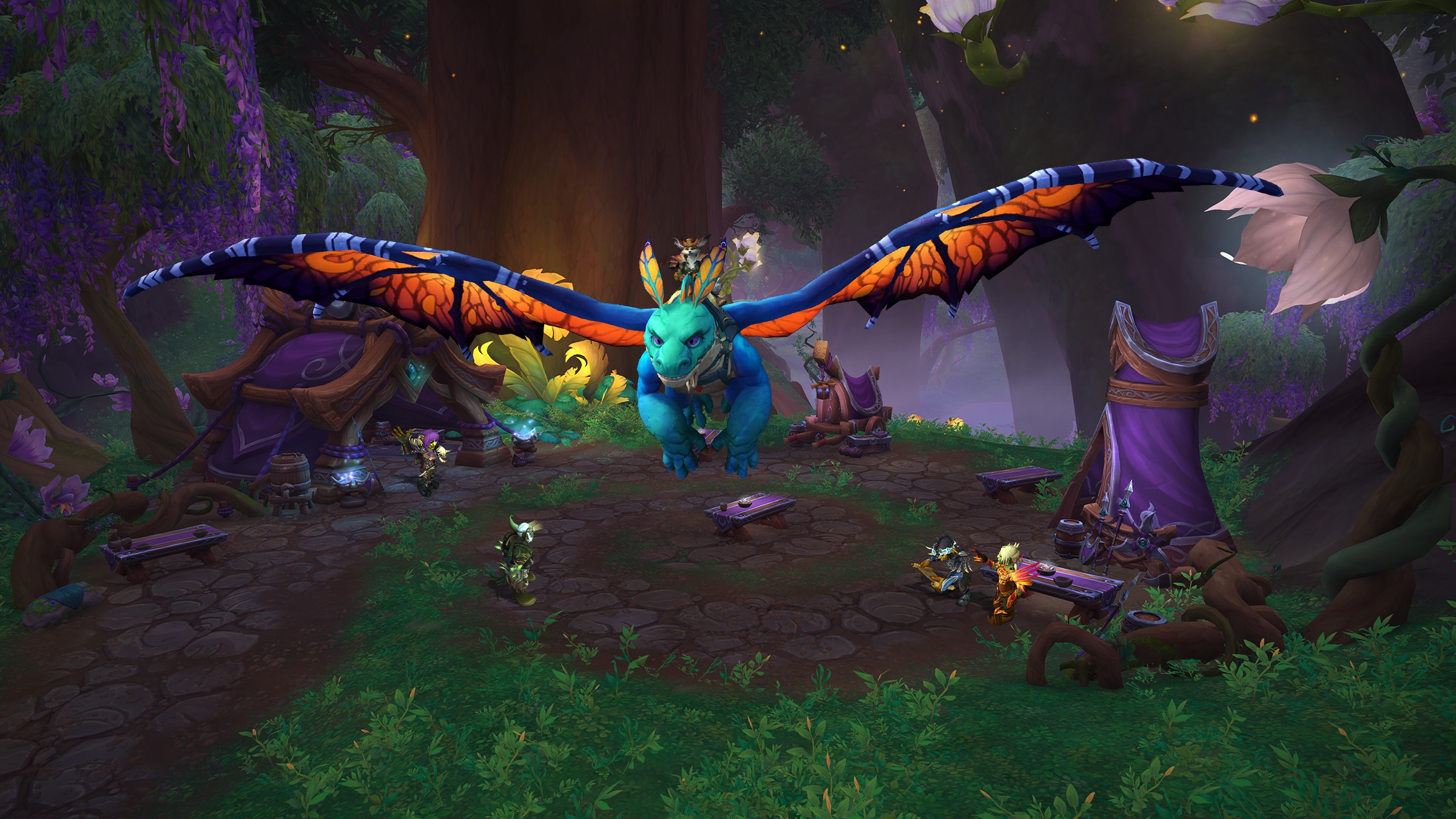This image, appearing to be a high-quality computer graphic from a fantasy video game, showcases a vivid, animated scene set in a mystical forest. Dominating the scene is a teal dragon with large, outspread wings that display a striking combination of blue and vivid orange underneath. The dragon, accented with orange and green antennae, is captured mid-flight, soaring above a quaint village of purple structures. This village includes a purple tent with a wooden frame, a purple tower, and several purple tables, suggesting a harmonious, unified design. Central to the village is a spiraled stone pathway, circled by lush vegetation featuring vibrant green grass, shrubs, and towering trees with a mix of green and purple foliage and drooping flowers. Scattered yellow leaves and a creamy white flower add to the idyllic setting. In addition, there's a sense of enchantment enhanced by a faint mist enveloping the tree trunks and branches in the background, contributing to the overall fairytale atmosphere.